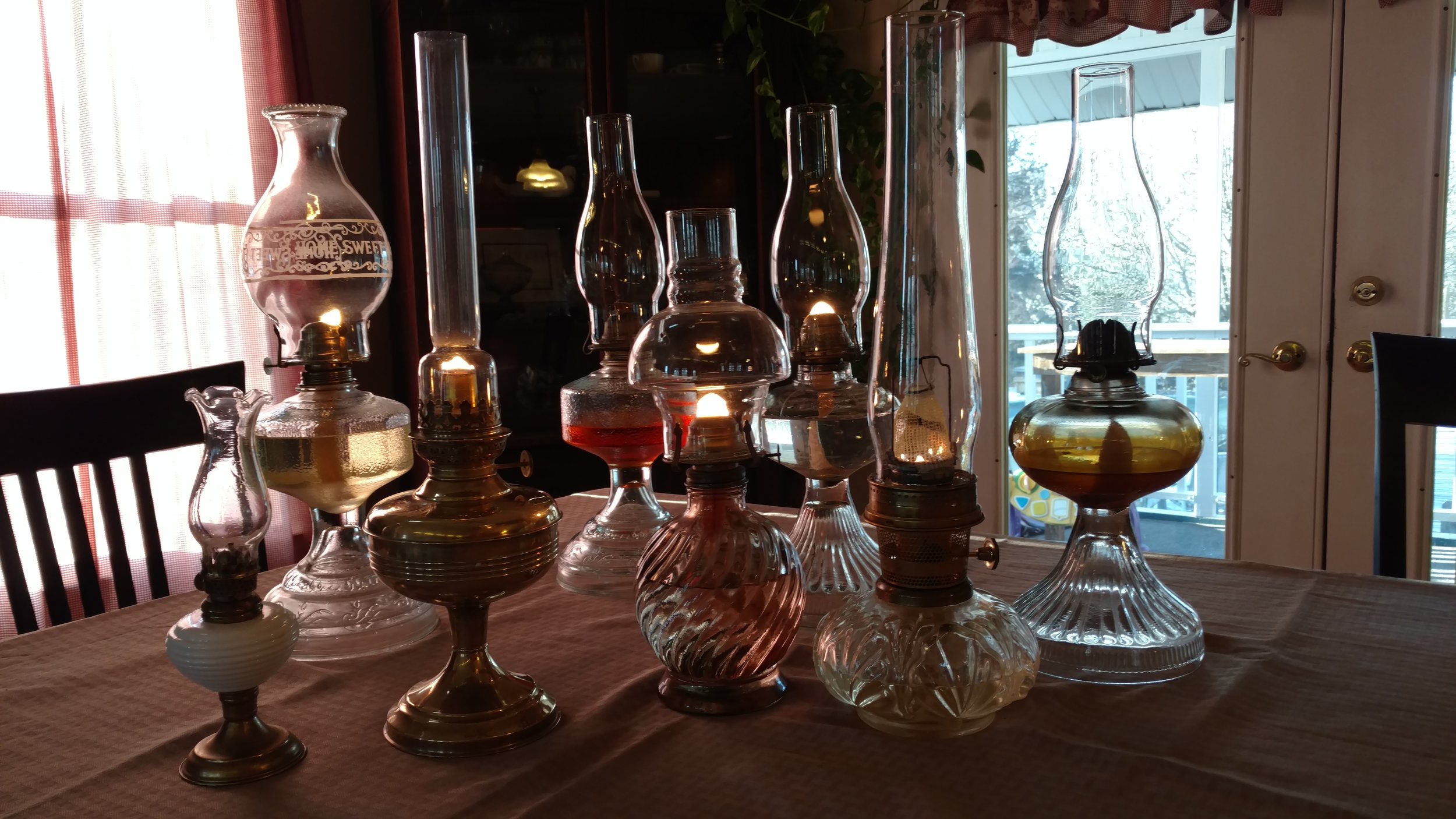In this indoor scene, a rectangular wooden kitchen table is prominently featured, adorned with a white tablecloth. Surrounding the table are brown wooden chairs, one visibly placed at the end and another partially visible on the side. The background showcases a double door with a full-length glass insert, leading to an outdoor patio and awning. To the left of the door, there is a window draped with translucent red curtains.

Resting on the table is an impressive collection of 10 to 15 antique lanterns, primarily kerosene hurricane-style lamps, varying in height and design. These lamps feature a distinctive glass chimney on top and a reservoir base at the bottom. The glass elements come in diverse colors, including clear, yellow, brown, and red, and some lamps exhibit textured glass. Occasionally, candles can be seen inside them. The tallest and largest lamp boasts a particularly widened base and reservoir, emphasizing its prominence within the collection. Collectively, they present an intriguing array of vintage illumination, contributing to the rustic and nostalgic ambiance of the room.